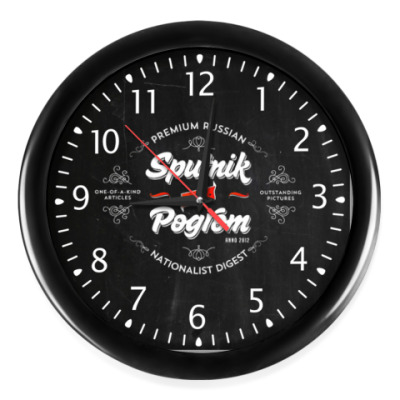The image depicts a clock with a black face known as the Sputnik Pogrom. It features classic white indicators in a circular pattern, with numbers from 1 to 12 marking the hours. The clock has three hands: the hour and minute hands are black, while the second hand is a thin, vivid red. At the top, in small white text, it reads "Premium Russian," with "Sputnik Pogrom" in larger white letters centrally positioned. Below the center, above the 6 o'clock mark, is the label "Nationalist Digest." Flanking the 9 and 3 positions are indistinct logos, difficult to discern due to their small size. The clock's design includes finer details, such as four smaller tick marks between each hour, with a slightly brighter mark indicating each hour position. The time shown is two minutes past nine.